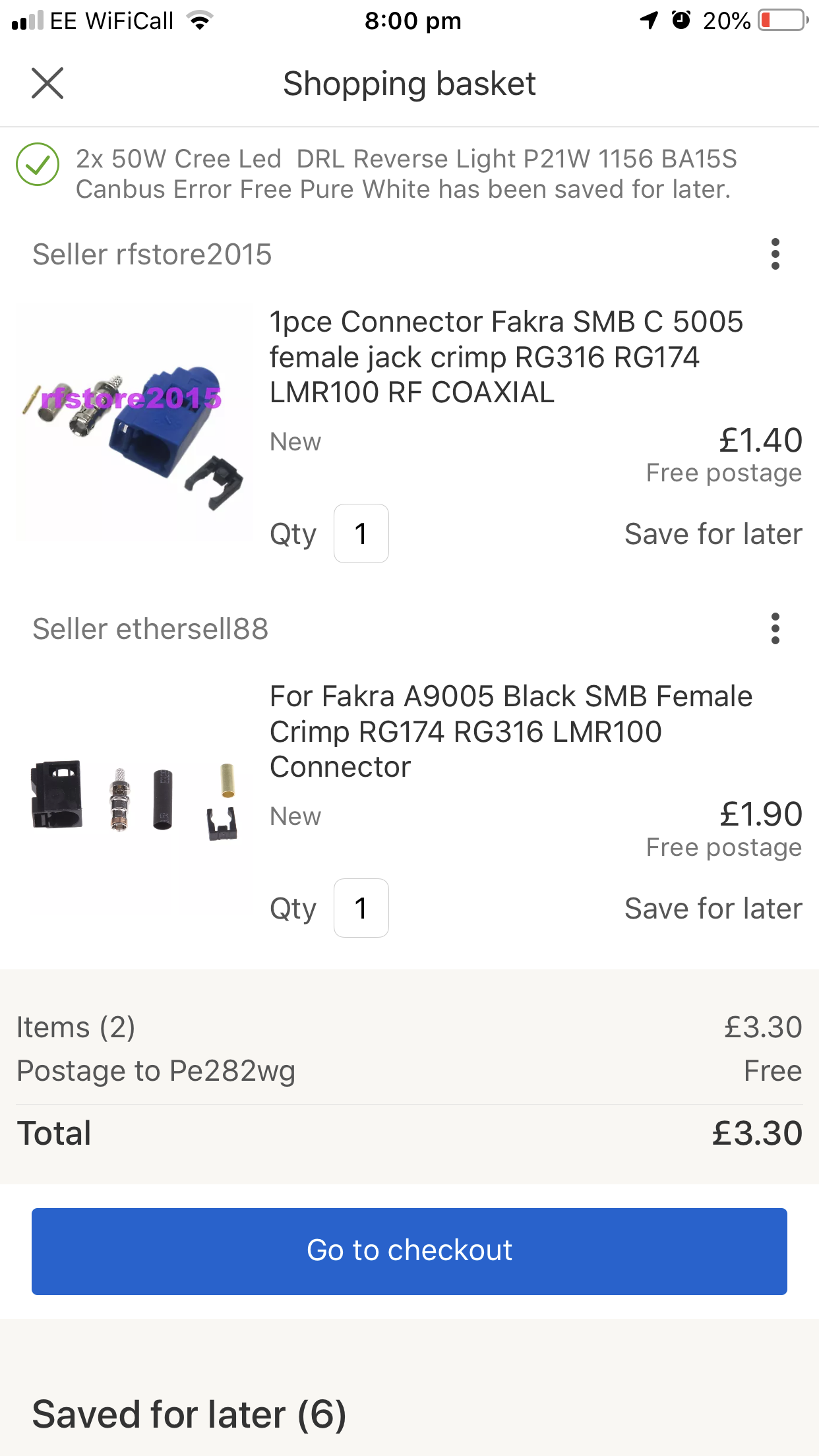This is a screenshot taken from a mobile phone displaying a shopping cart interface from an online marketplace. 

At the very top of the screen, there are various status indicators: the mobile signal strength is shown with two out of five bars filled, and the carrier is listed as "EE". The Wi-Fi calling feature is active, indicated by the label "Wi-Fi call" and Wi-Fi signal bars, which also show two out of four bars filled. The current time is displayed as "8:00 PM". On the far right, icons include a send arrow pointing upwards, a clock, and a battery symbol showing 20% remaining with a red indicator.

The shopping cart section features two items. In the middle of the screen, a shopping basket icon is displayed. To the left, an "X" icon is visible, likely for removing an item, separated by a thin line. Below this, a green check mark indicates an in-stock item labeled "2X5W Cree LED DRL reverse light P21WL 1156BA15S" sold by "RF store 2015". An image of the product is shown alongside essential details. The listed quantity is "1", and the price is "1.40" in either pounds or euros, with free postage. Below this, an option to "Save for later" and additional seller information reads "S for sell 88".

Further down, another item is listed: "Fakara A900 black SMB female", noted as a connector. It includes a media image and is sold by the same seller as the previous item. The quantity is also "1" and the price is "1.99" in either pounds or euros, with free postage available. The option to "Save for later" is again provided.

At the bottom, there is a summary of the total cost and a blue rectangular button labeled "Go to checkout". Below this, there's another "Save for later" option listing six items saved for future consideration.